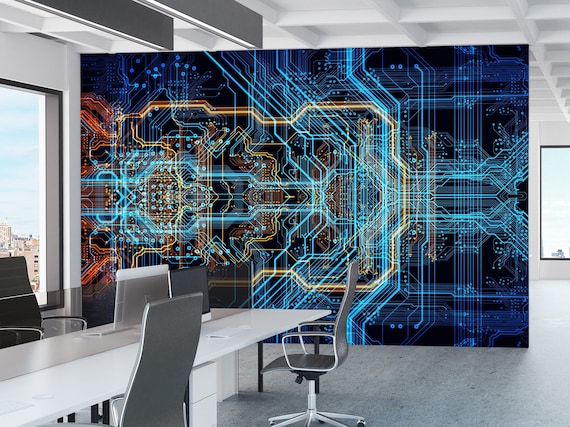The image captures a very modern and sophisticated conference room. At its center is a long, narrow rectangular table that is predominantly white with a taupey cream color blending in. Intriguingly, a sleek glass divider runs through the middle of the table. Surrounding the table are elegant gray chairs with high, narrow backs and white arms, featuring wheels for easy movement. Notably, two computer monitors are positioned on either side of the divider.

The room's aesthetic emphasizes white and gray tones, with a very minimalist and clean look. A large plate glass window offers a view of the blue sky and adjacent buildings, enhancing the sense of openness. The backdrop is striking: a mural depicting an abstract electric circuit board pattern with a dark blue background. This mural is adorned with vibrant lines in neon blue, orange, yellow, and red, creating a crowded and dynamic visual impact.

In the room's background, you can observe details such as white ceiling squares and another plate glass window, adding layers of depth and light to the overall setting. The combination of modern furniture and vibrant artwork makes this conference room both functional and visually stimulating.